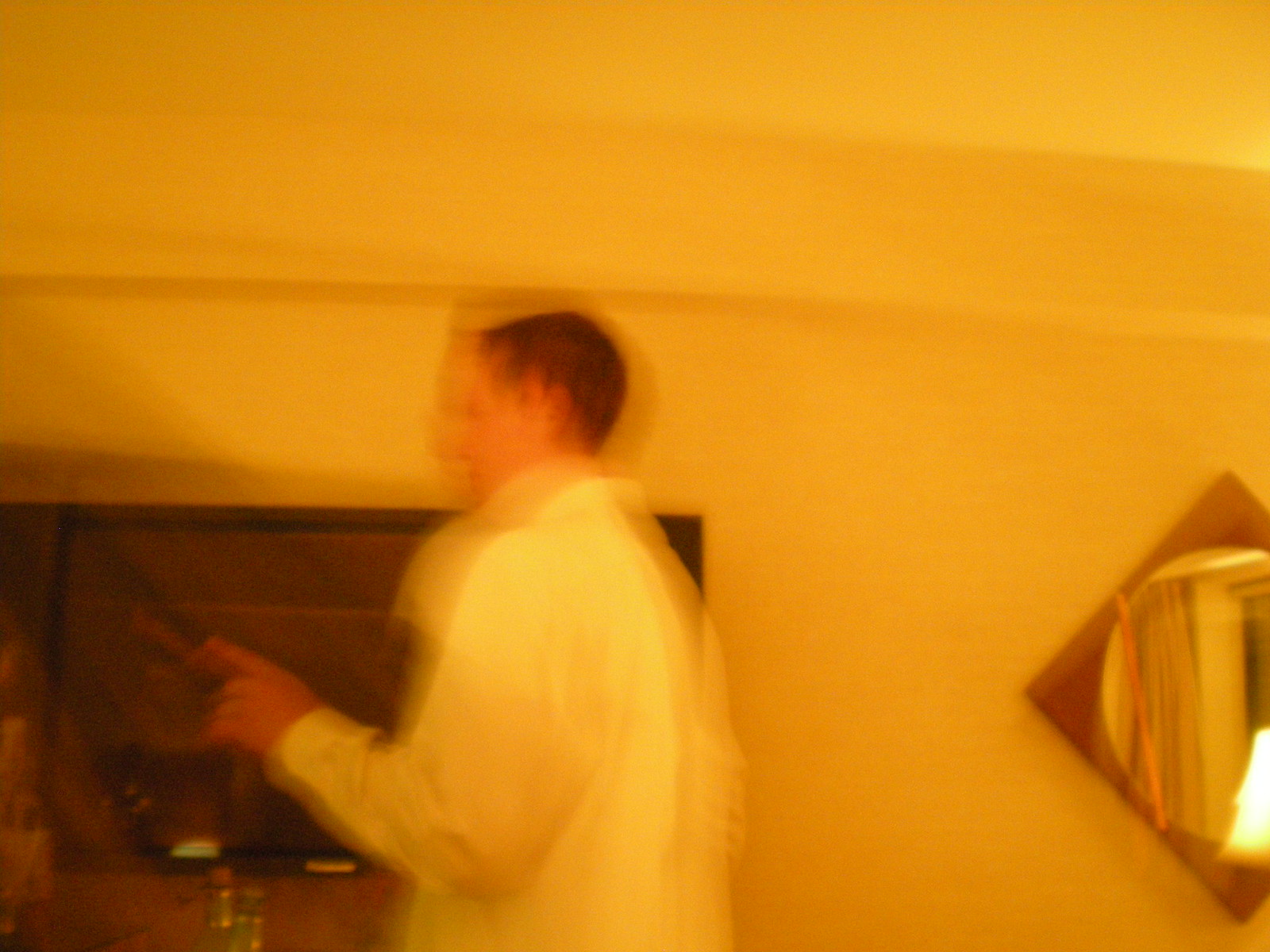The blurry and miscolored indoor photo captures the side profile of a man with short brown hair, standing slightly to the left in the image. He is wearing a baggy white shirt and appears to be pointing forward with his left hand, adding an air of explanation or instruction to the scene. In the background, a white wall frames a wood shelf, while a glass bottle with a cork is visible just below his hand. Noteworthy elements in the surroundings include a diagonal diamond-shaped framed mirror towards the lower right and possibly the edge of a lamp. The overall lighting casts a bright yellow wash over the scene, suggesting it might be taken at nighttime under warm artificial light. Despite the intentional or accidental blurriness, the image centers on this man who seems engaged in some sort of explanatory action, possibly engaging with an unseen audience.